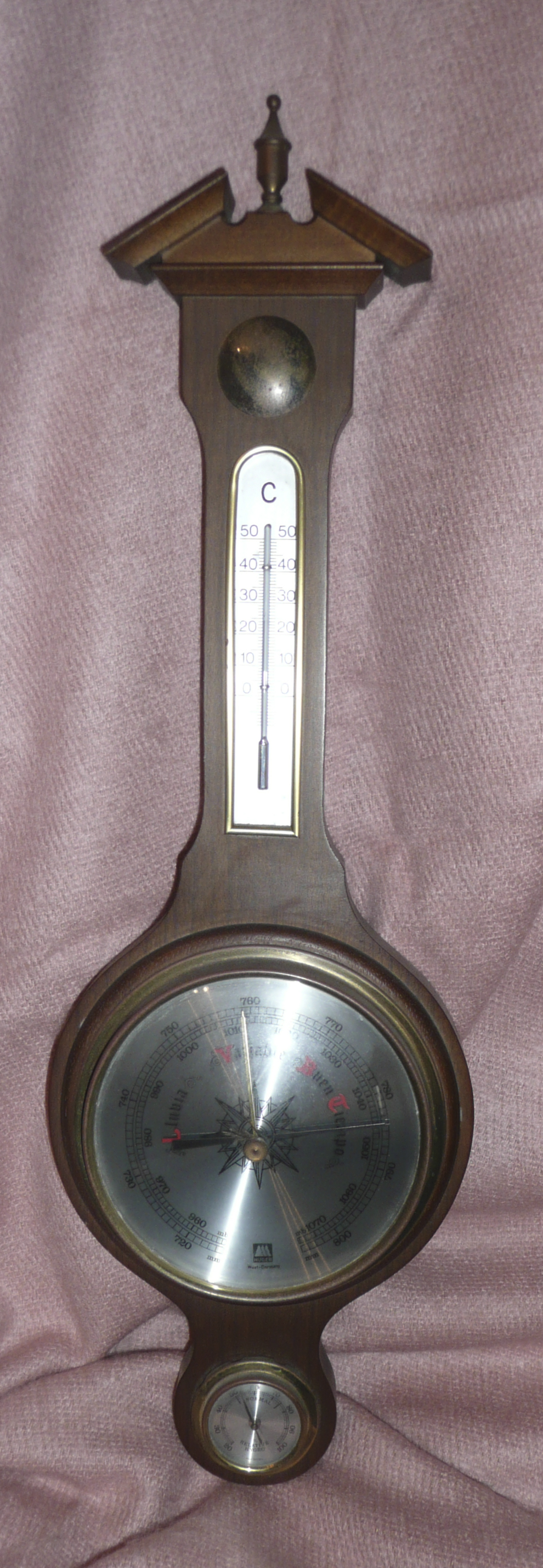This image features an elongated, slanted clock structure, adorned with multiple decorative elements. At the pinnacle of the structure, it tapers into a pointed tip. Positioned at one end, there is a large, circular clock face. Below this clock, the structure widens to reveal a prominent black circle. Directly beneath the black circle is a silver thermostat, marked by a "C" inscribed at its top. The light striking the thermostat creates a noticeable glare, highlighting the metallic sheen of the device. Further down, the structure includes a massive silver circle, which also catches the light, adding to the intricate design. At the very bottom, a smaller circular clock face completes the composition, enhancing the clock's unique and detailed aesthetic.